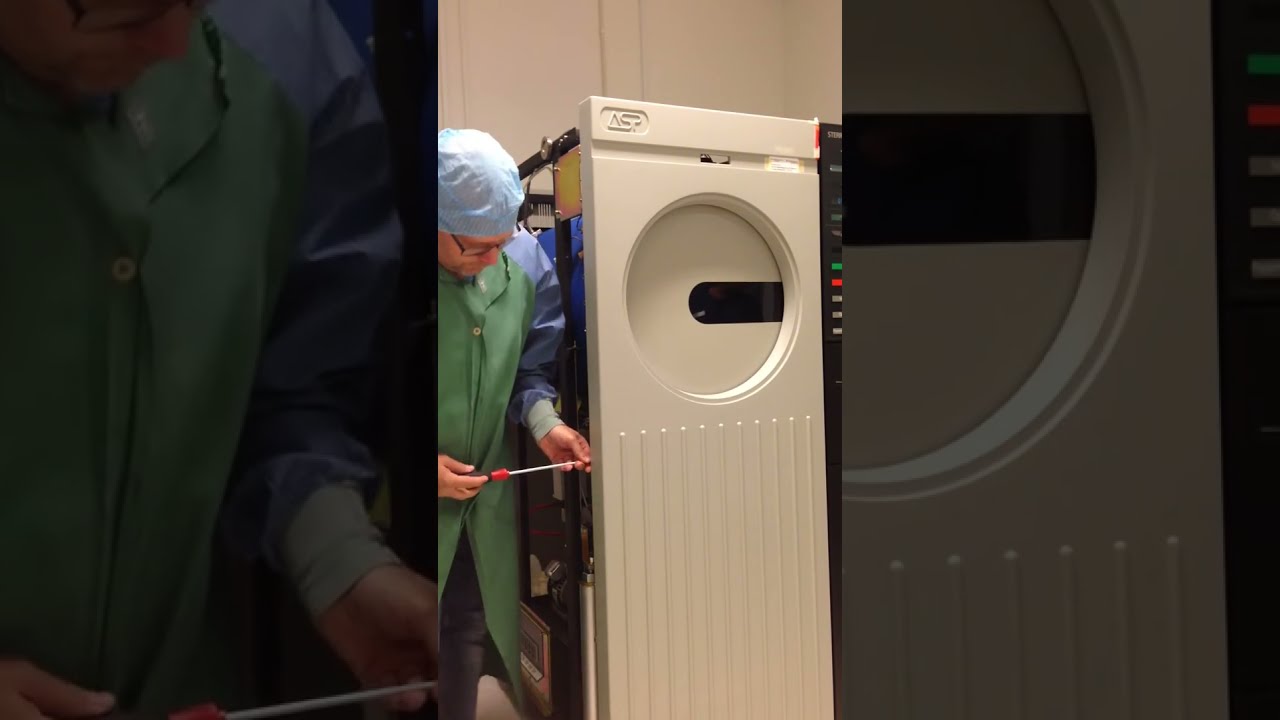The horizontally aligned rectangular photograph features a thick, solid black border framing a centrally placed vertical rectangular image. This central photograph portrays a worker in a medical setting, identifiable as a doctor by their attire. The doctor, positioned in the lower left corner, is bending over, obscuring their face, and is wearing eyeglasses along with a white fabric paper hat, a green protective shield around their neck, a green shirt underneath blue scrubs. 

Adjacent to the doctor on their right is a substantial medical device, identifiable by its white front paneling, a black side panel with an array of colored buttons, and a prominent circular area that resembles the tunnel entrance of an MRI machine. A logo with the letters "ASP" is visible on the device. Extending into the background is a blue cylindrical component of the machine, interconnected with various wires or tubes, and framed by black metal.

The background is dominated by a white wall, enhancing the clarity and realism of the clinical setting captured in the photograph. The image is detailed and precise, highlighting the specialized nature of both the equipment and the professional attending to it, encapsulating a moment of focused medical activity.